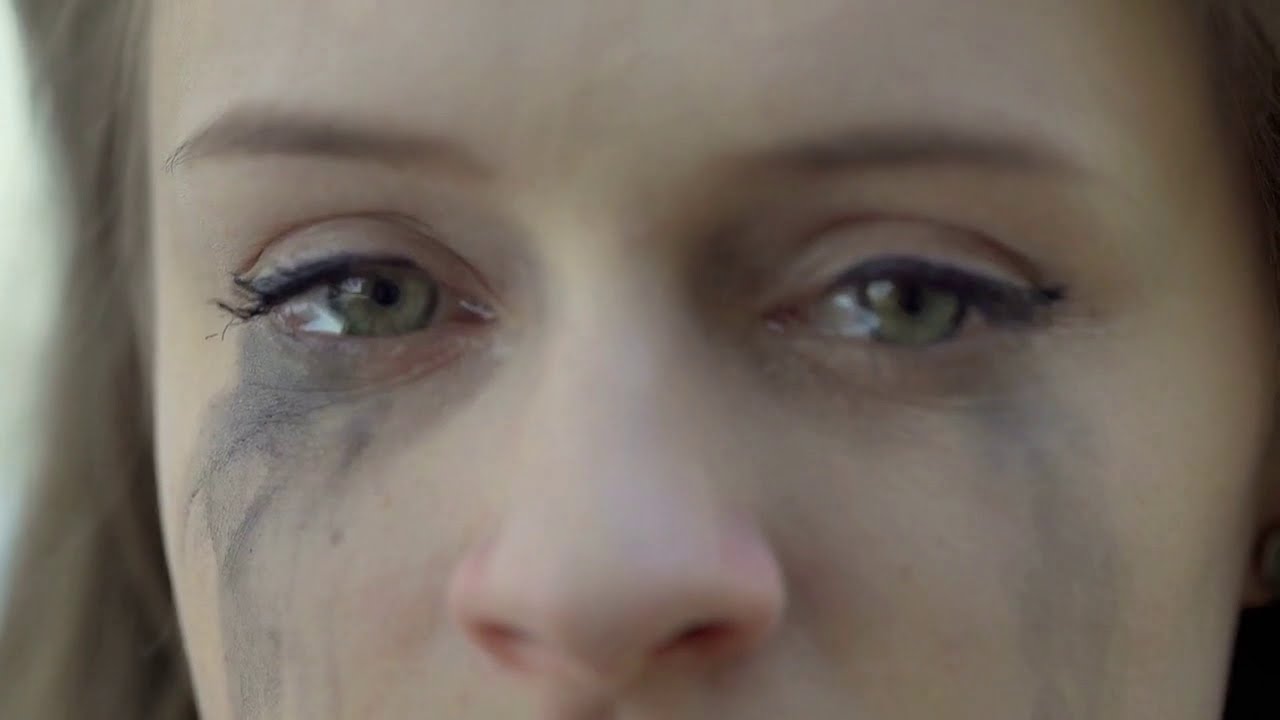This horizontal, landscape-oriented color photograph presents an extreme close-up of a woman's face from just below her nose to the midsection of her forehead. Her medium to dark brown hair frames a sorrowful expression. Mascara and black eyeliner have run down her cheeks, forming black streaks beneath her hazel or gray-tinged eyes, evidence of her recent crying. Tears still glisten in her eyes, further reddening her nose. The image focuses more clearly on her right eye and cheek, while her left side appears slightly blurred. Her penciled-in brown eyebrows and realistic, photographic representation intensify the emotion captured in the photo, suggesting she is in her 20s or 30s.